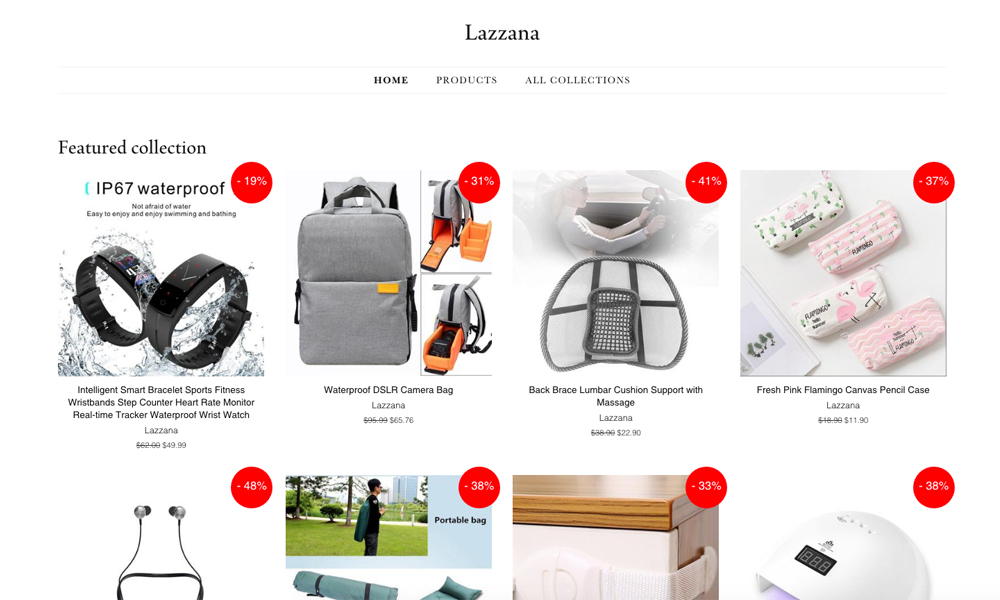Featured on the Lazana Lazana website (spelled L-A-Z-Z-A-N-A), the image captures the homepage adorned with drop-down menus labeled "Home", "Products", and "All Collections". Below these menus, the site showcases eight clickable product boxes arranged neatly in two rows of four.

Zooming in on the top row, the first box highlights the "Featured Collection" with an IP67 waterproof sports fitness wristband. This versatile wristband functions as a step counter, heart rate monitor, and real-time tracker, all while being waterproof. It is available in black and boasts a 19% discount, currently priced at $49.99.

Adjacent to it, the second box presents a waterproof DSLR camera bag. The third box offers a back brace with lumbar cushion support that includes a massage feature. The fourth box on the top row showcases a fresh pink flamingo canvas pencil case.

In the bottom row, starting from the left, the products displayed include what appears to be wireless earbuds, though the full description is cut off. Next to that is a portable yoga bag. The third product in this row is a childproof drawer lock. Finally, the last box on the right seems to feature a device emitting a purple light, likely a nail dryer.

Overall, the image gives a detailed glimpse into the diverse range of products available on the Lazana Lazana website.